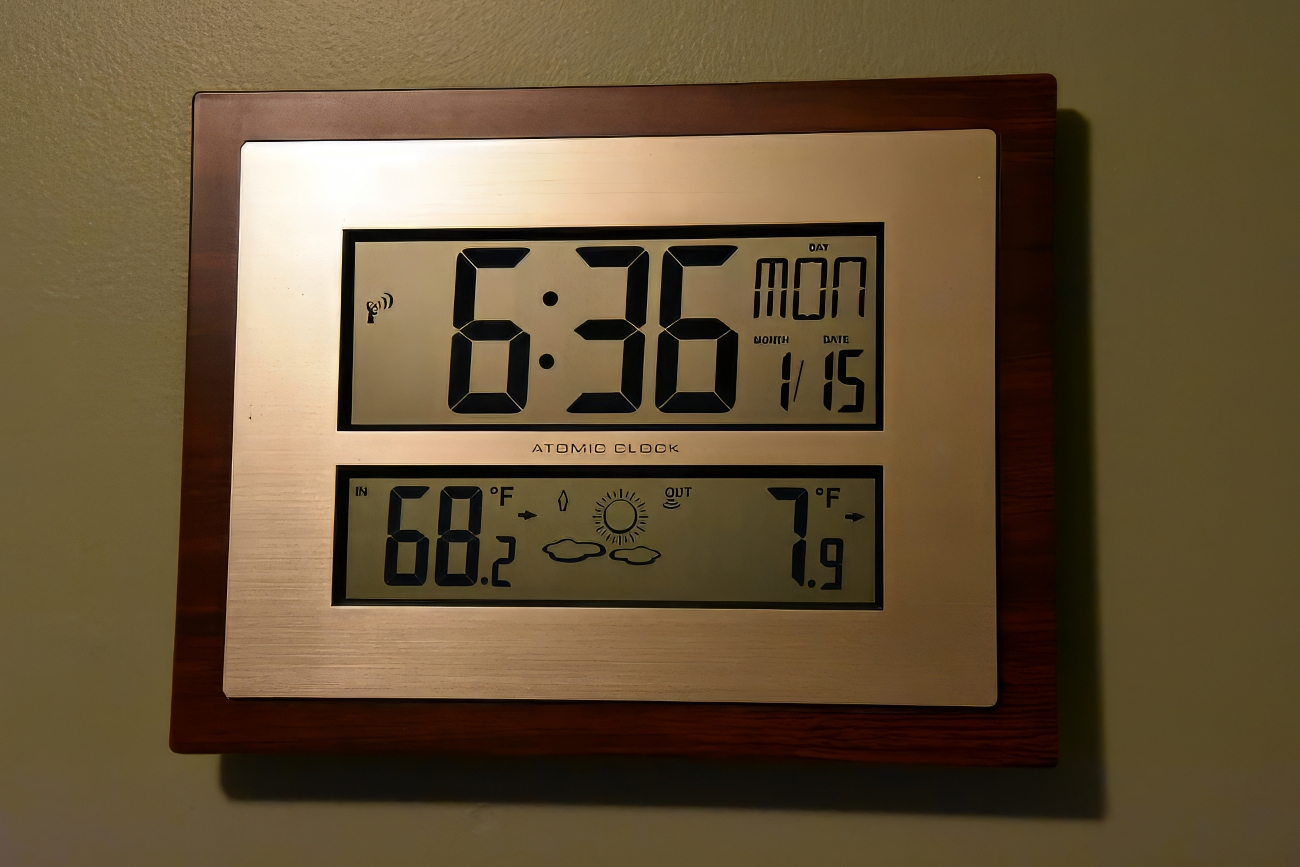This is a horizontal photograph featuring a digital clock prominently displayed against an olive-painted wall. The clock, encased in a dark wood rectangle frame with a brass front, takes up most of the image. It is mounted on the wall, and the light source emanating from the upper left casts a distinct shadow of the clock slanting down to the right.

The clock has two main LCD screens. The top screen, larger than the bottom, displays the current time as 6:36. Above the time, "Atomic Clock" is inscribed, indicating that it receives its time updates from an atomic clock source. A small radar dish icon with wave lines appears on the left side of this screen. Additionally, the day and date are shown as Monday, January 15.

The smaller bottom screen seems to provide weather information. It displays a temperature of 68.2 degrees Fahrenheit alongside an icon depicting clouds and the sun. Beneath the term "Out," emphasized with lines, it shows another temperature reading of 7.9 degrees Fahrenheit.